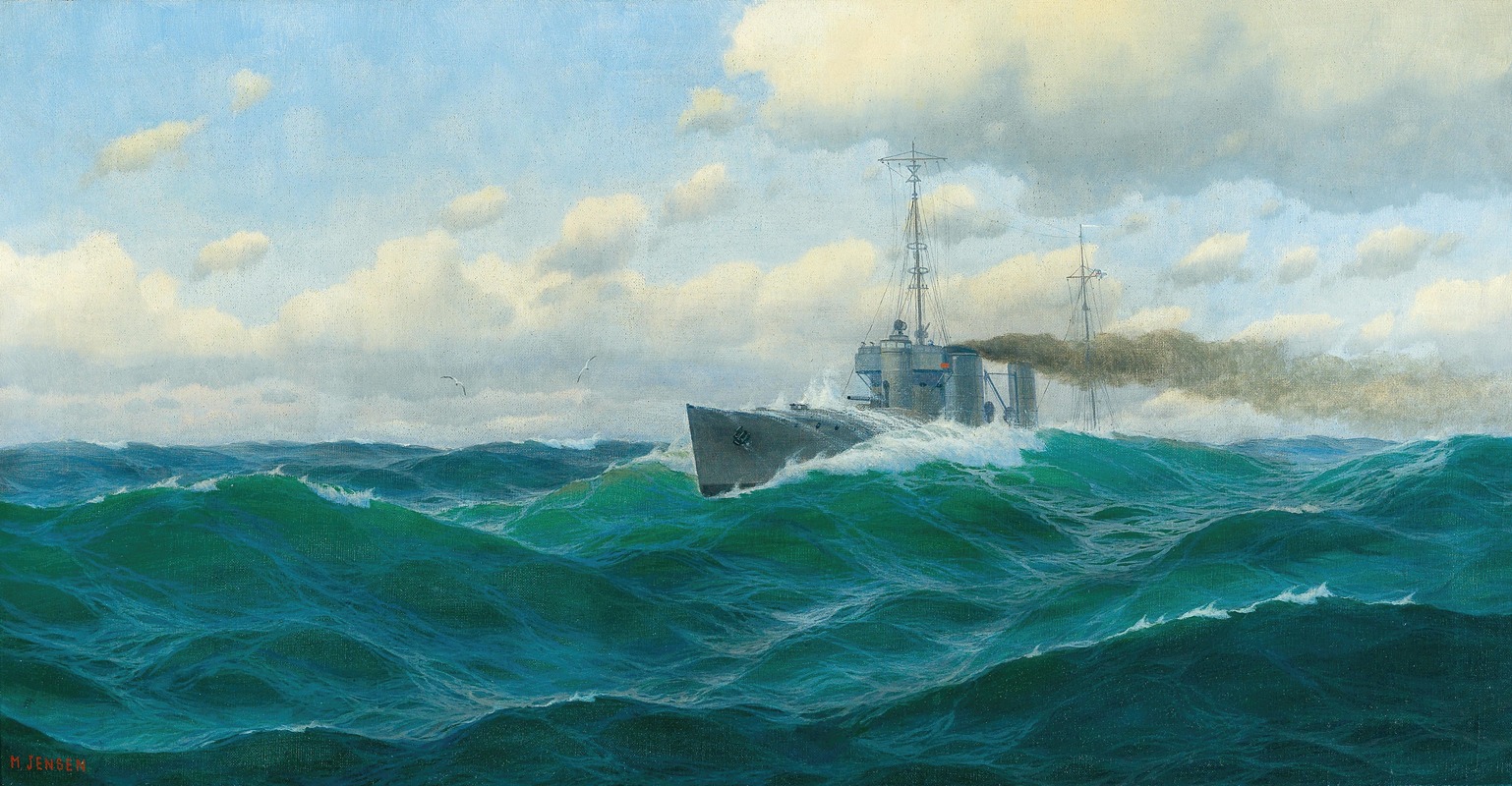The image is a detailed, rectangular landscape illustration, approximately two and a half to three times wider than it is high, depicting a large gray military ship caught in a choppy sea. The sky above is a bright blue, peppered with numerous fluffy white clouds. The majority of the bottom half of the image is dominated by the turbulent ocean, with medium blue to greenish-blue waves capped with white foam.

The ship, likely a battleship, is centrally positioned, slightly to the right, and appears elongated with roughly half of its structure visible above the water. The vessel is navigating through the sizeable waves, creating an impression that its pointed nose is slicing through the water without sustaining any damage. The ship tilts subtly to the left, an effect amplified by the way the sea laps against its hull.

Several cylindrical smokestacks are visible atop the ship, from which dark gray smoke billows backward. Two masts, resembling telephone poles, rise from the ship's deck, though they lack any sails. The composition and perspective suggest a dynamic scene, with the battleship forging ahead through the rough, greenish sea under a blue sky filled with clouds. The image is devoid of any visible text or additional objects, focusing solely on the ship and its maritime journey.